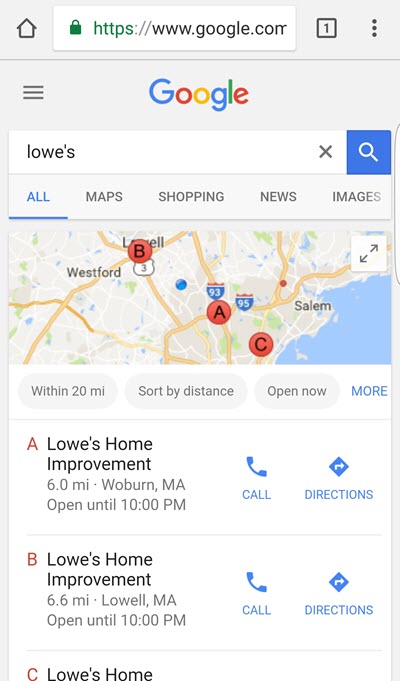The image depicts a smartphone displaying a Google search results page for "Lowe's Home Improvement" in the Massachusetts area, likely targeting "Woburn" and "Lowell." At the top of the screen, the familiar Google logo is visible, followed by a search bar with the query for "Lowe's Home Improvement." Below the search bar, there are tabs labeled "All," "Maps," "Shopping," "News," and "Images."

The main section of the screen shows a map with markers labeled A, B, and C, indicating different Lowe's locations. Underneath the map, there are filter options to sort by distance or open status, and a blue link labeled "More." Specifically:

1. Location A lists "Lowe's Home Improvement," situated 6 miles away in Woburn, Massachusetts, and notes that it is open until 10 PM. It includes buttons for "Call" and "Directions."
  
2. Location B also specifies "Lowe's Home Improvement," located 6.6 miles away in Lowell, Massachusetts, with the same closing time and similar action buttons.

3. Location C mentions "Lowe's Home Improvement," but the full details are not visible at the bottom of the screen.

This Google search image captures a typical smartphone interface for finding nearby Lowe's stores in the Massachusetts area.